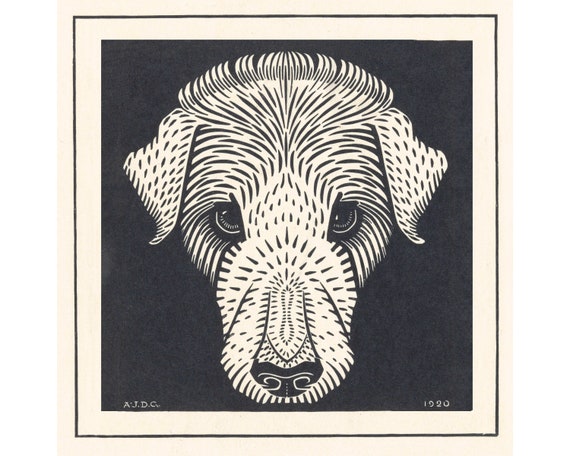This captivating image is an abstract, artistic illustration of a dog's face, rendered in black and white. The dog's head is centrally positioned on the black background, giving prominence to its deep, dark eyes and solidly filled-in black nose. The rest of the dog's facial features, including its ears and the bridge of its nose, are suggested with delicate black lines that convey the texture of individual hairs, while the head appears to be emerging from a white surrounding area. There's a distinct thin black border framing the entire image. At the bottom left of the picture are the initials "A.J.D.C.", likely those of the artist, while the bottom right corner bears the year "1920", possibly marking the creation date. This image, reminiscent of a lithograph, impressively blends solid, well-defined marks with subtle lines, capturing the essence of the dog in a strikingly minimalist yet detailed manner.